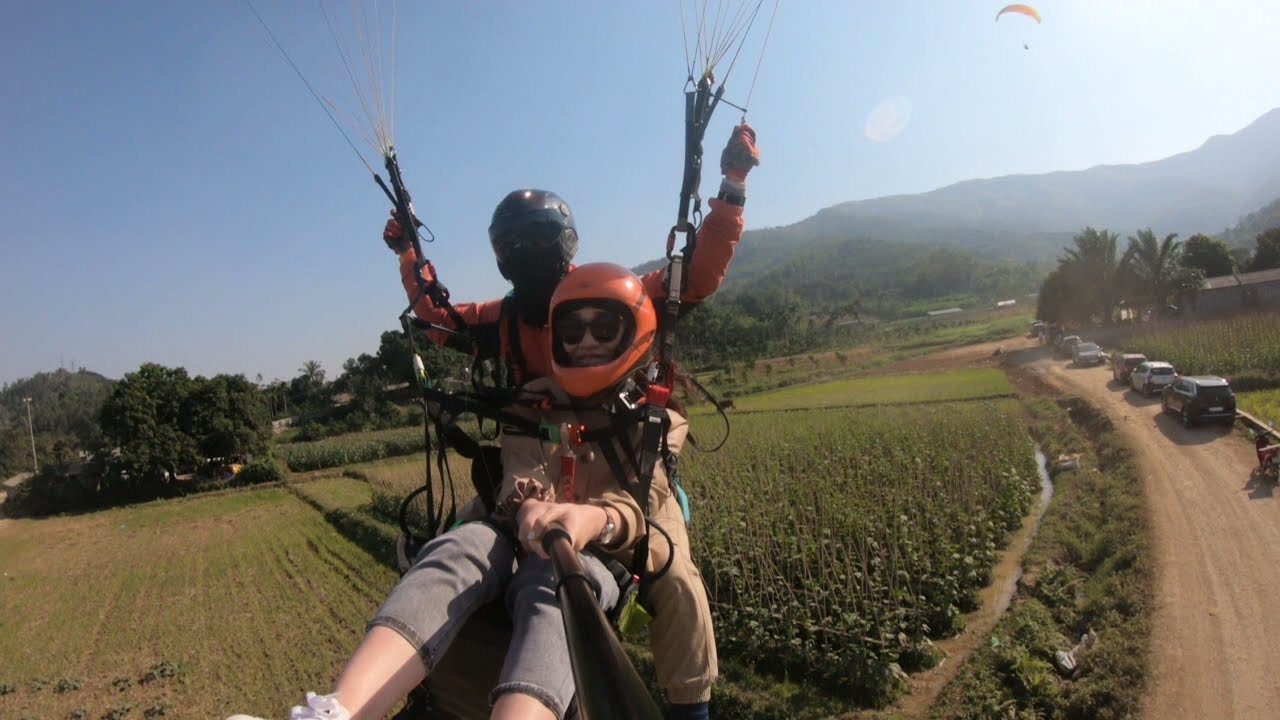In this vibrant and detailed outdoor photograph, we see two people paragliding in what appears to be a tropical farm field landscape. The scene captures a woman and her instructor, both about 20 to 30 feet from landing. The woman, dressed in grey capris, white shoes, an orange helmet, and black sunglasses, is holding a selfie stick with both hands, capturing this thrilling moment. Her legs are raised as they descend, and she is strapped securely with safety harnesses. Behind her, the instructor is in control of the parachute, wearing a black helmet, mask, an orange t-shirt, and brown trousers. The background features lush greenery, a combination of palm trees, mountains, hills, and a road strip with parked cars. The clear blue sky and distant sun rays illuminate the scene, and another parachuter can be spotted far off in the top-right corner of the image. The entire composition, which is a horizontal rectangle, highlights the vibrant colors of orange, red, brown, green, grey, and blue, emphasizing the dynamic and picturesque setting of this adventurous moment.